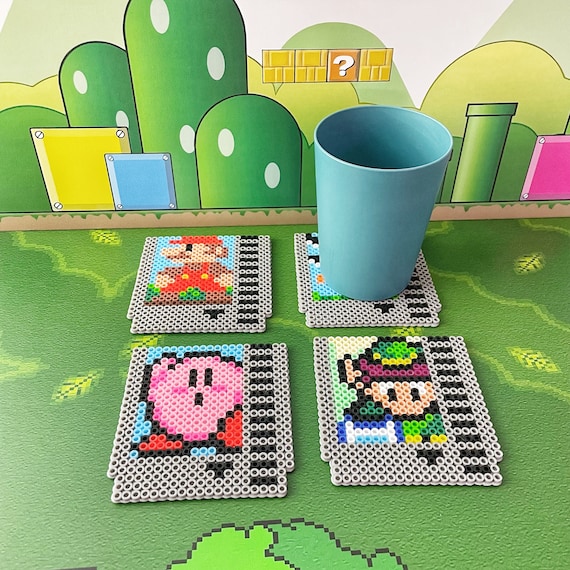In this image, we see a detailed homage to the classic Super Mario Bros. video game series. The backdrop features a wall decorated to resemble a stage from the Mario games, primarily using green pixel art to mimic the cartoony bushes, complete with green arches dotted with white spots. Centrally, on this paper background, are four squares: the first two and the last square look like gold bricks, while the third square displays the iconic question mark block. 

Further enhancing the Mario theme is a big green tube sprouting from the bottom of the wall, reminiscent of the pipes Mario frequently travels through. Adjacent to the tube is a pink square. 

In the foreground, situated on a green surface, are four coasters that resemble old-school NES cartridges created from ironed pony beads. The details on each coaster add to the nostalgic charm: the top left coaster features Mario in his red attire and distinctive mustache. The coaster in the bottom left showcases Kirby, the pink puffball character. The bottom right coaster depicts Link from The Legend of Zelda series. Unfortunately, the image on the top right coaster is obscured by a blue cylindrical cup, which appears to be empty.

The table setup, possibly in a breakfast nook area, marries functional decor with nostalgic nods to beloved video game characters and artifacts, capturing both the whimsy and artistry of the Mario Bros. universe.